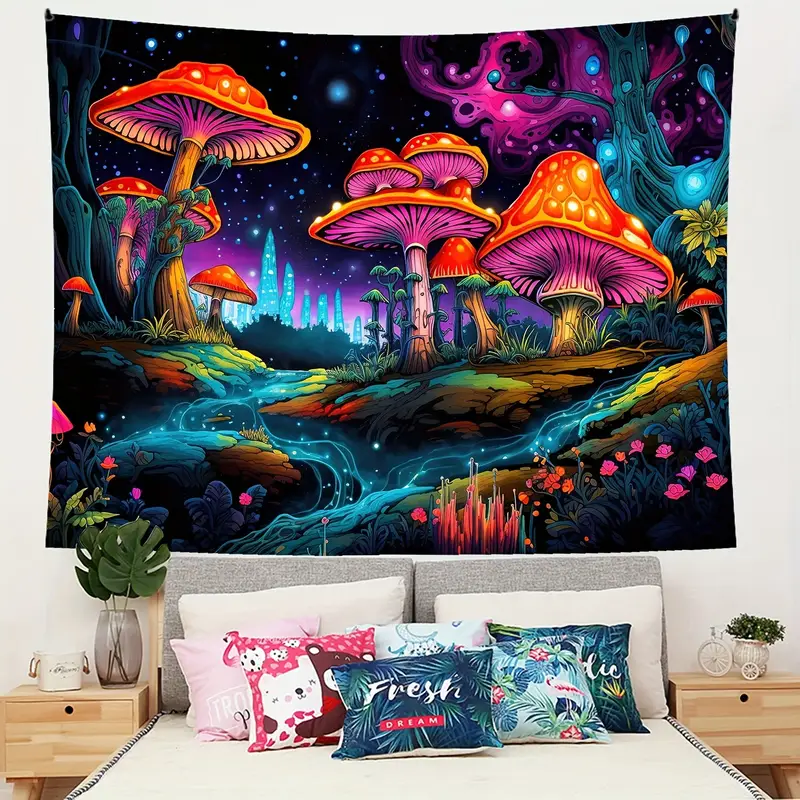The image depicts a cozy bedroom featuring a pristine white bed adorned with a variety of pillows, including two large gray pillows at the back, two large white pillows in front of them, and an assortment of colorful throw pillows. Notable throw pillows include one with "Fresh Dream" printed on it, a pink and spotted pillow featuring hugging bears, and a more forest-themed pillow among others. The bed is covered with a white blanket.

On either side of the bed are wooden end tables; the left one accessorized with a vase containing a few large green leaves and a small white bucket, while the right one features a small plant inside a miniature bicycle or wagon.

Prominently displayed above the bed is a large, vibrant, and trippy wall hanging. This tapestry, set against a black night sky background, showcases a surreal, almost psychedelic landscape. At the center of the tapestry, towering mushrooms with bright orange caps and red stems rise to tree-like heights. The scene is further embellished with a vivid blue river flowing through lush greenery dotted with colorful flowers and other plants. Scattered across the sky are light blue star-like dots, adding to the dreamlike quality of the image. The tapestry is secured to a light gray wall, forming a striking focal point in the room.